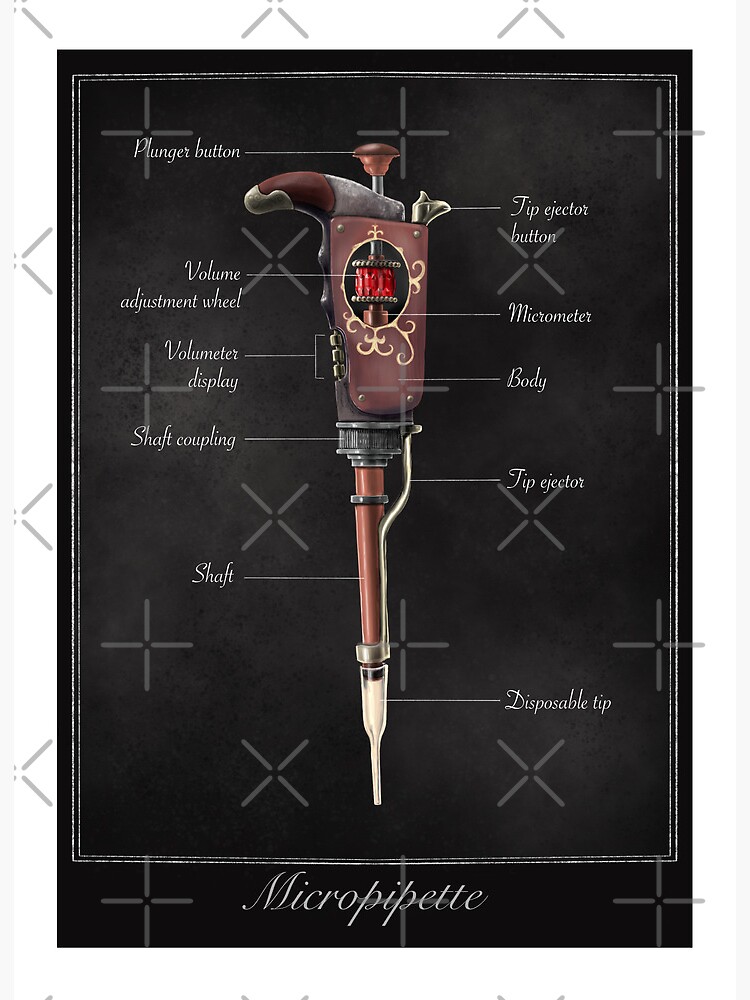The image depicts a detailed illustration of a micropipette against a black background adorned with X and plus signs. The micropipette, commonly used in laboratories for precise liquid measurement, is meticulously labeled with its various parts. At the top, the plunger button, resembling a small brown knob, sits alongside a tip ejector button. Below, on the left side, the volume adjustment wheel is marked, notable for its red color with metallic accents, adjacent to the volume meter display. The micrometer and the main body of the device are indicated on the right. Moving down, the shaft coupling connects the handle to the shaft, which is described as a brown tubular form. Along the shaft runs a metallic bar, identified as the tip ejector. At the bottom of the device, labeled with a straight line pointing right, is the disposable tip, marked in white and designed to be replaceable. The entire image is framed within a light gray border, with "micropipette" written in italicized light gray text at the bottom, confirming the identity of the device.